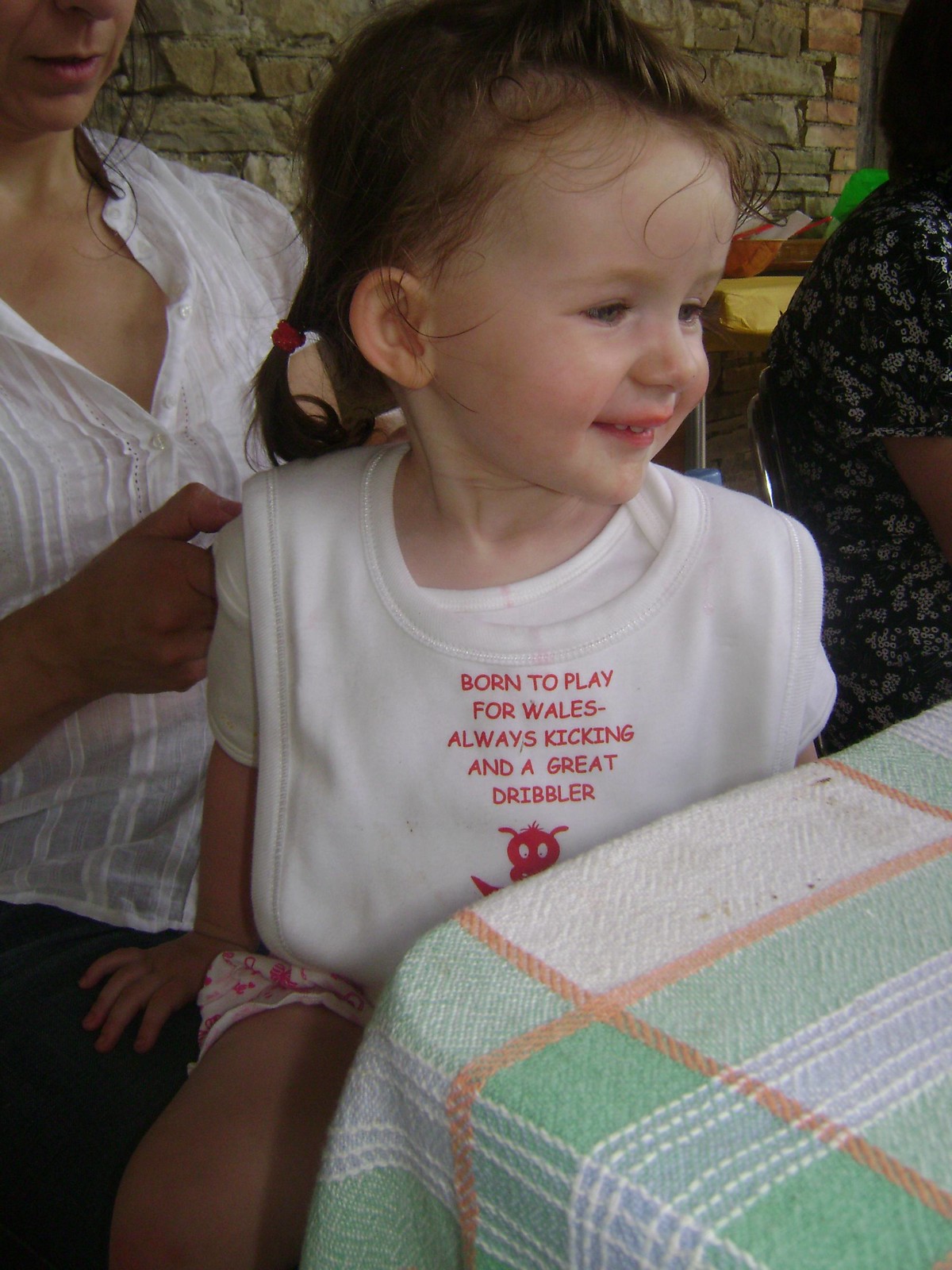The image captures a sweet moment of a very young girl, likely around two to four years old, sitting on a woman's lap at a table. She wears a white baby bib with red text reading, "born to play for whales always kicking and a great dribbler," accompanied by a partially obscured cartoon-like graphic of an animal. The girl has white complexion and her hair is tied with a red hair tie. She gazes off to her right with a pleasant expression, while the woman holding her, who has a white shirt and denim pants, supports her at the corner of the checkered table. The tablecloth is a mix of green, orange, gray, and white stripes. Another woman, partly cut off from the frame, is seen to the right, wearing black clothing with white floral elements and having black hair. The background features a brick stone wall, completing the cozy and homely atmosphere of the photograph.